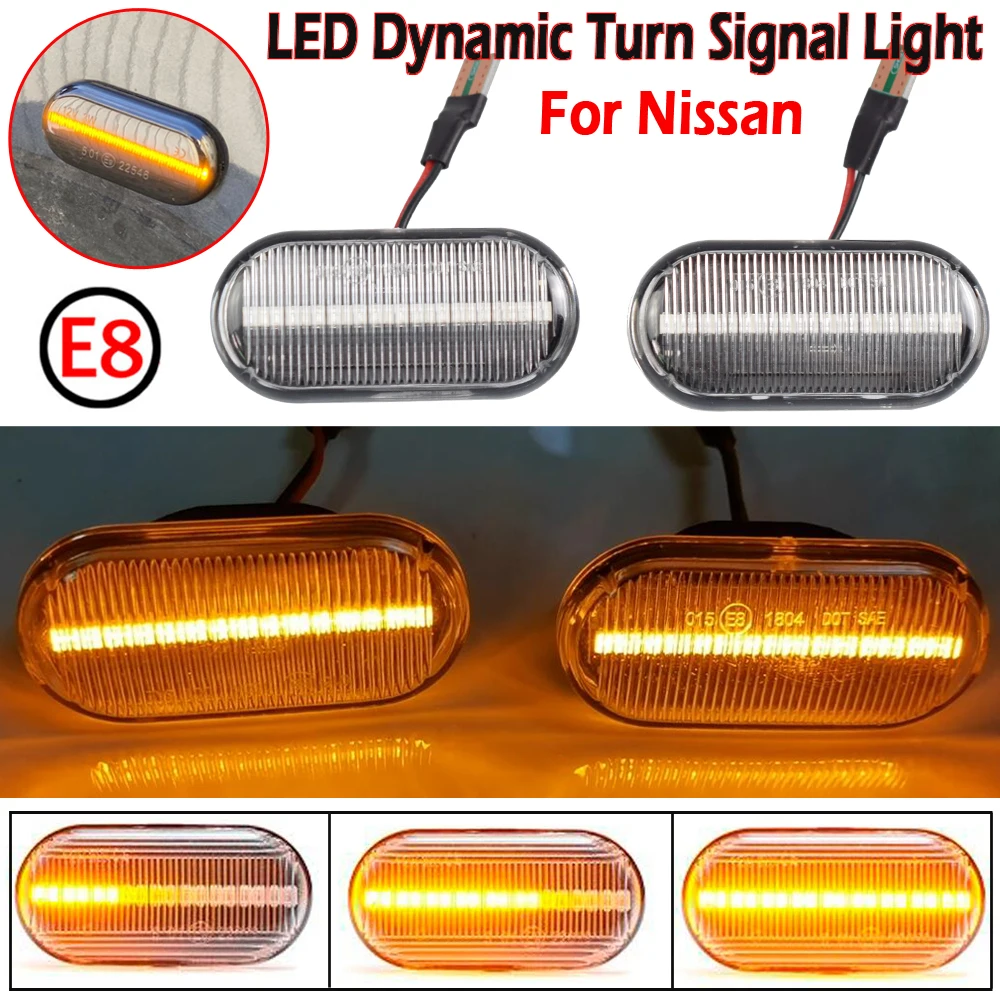This image appears to be an advertisement or product packaging for LED dynamic turn signal lights designed for Nissan vehicles. It prominently features a detailed depiction of the lights within their housings. The lights are oblong or capsule-shaped, reminiscent of a Tylenol capsule, and are made of white plastic with internal stripes and vertical ribbing. Each unit contains a bright LED strip, which can be seen functioning in various insets of the image.

At the top of the image, there are two LED light units with attached cables and a chrome or silver bezel around the external fixture. These lights are not illuminated or emit a white light only. An 'E8' circled in red font inside a black circle is also present in this section. Below, an inset shows these lights partially embedded in sand.

The middle section of the image displays headlights that are amber or orange in color with horizontal light stripes. These lights are labeled '015,' 'E8,' and '1804 DOT SAE,' emphasizing their compliance and specifications, which are permanently embossed into the plastic.

The bottom section of the image features three smaller lights side by side, showcasing different stages of illumination from a dynamic turn signal effect. The progression illustrates the light traversing from left to right, from a faint beginning on the left to full illumination of the entire LED strip on the right.

In total, there are eight individual light housings in the image, with the clear or white lights positioned at the top and the remaining amber lights spread across the middle and bottom sections.